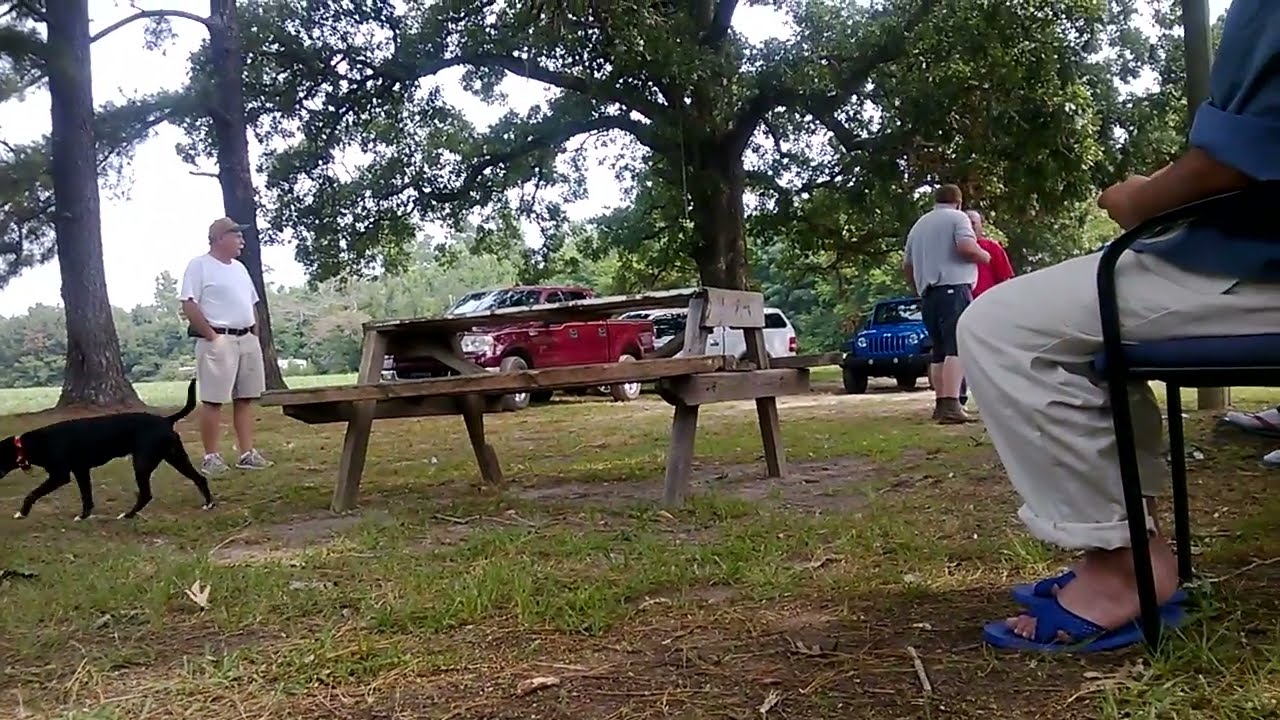In this vibrant spring or summer park scene, people are gathered around a picnic table seemingly engaged in a casual meeting rather than a meal. The main focus is a man standing with one leg up on the picnic table, pointing towards the right while holding some pieces of paper. Underneath the picnic table, a black dog with a red collar sniffs the ground. In the foreground, near the camera, a person sits in a possible folding chair, distinctly dressed in white pants, a blue shirt, and blue sandals. To the left, another man stands in creamish shorts, a white top, and a baseball cap, looking in the same direction as the man at the table. The setting features green grass mingled with patches of exposed dirt and is framed by a large tree and a distant line of trees. Cars are visible in a sandy gravel parking lot beneath the large tree, illustrating a typical picnic park scene on a bright day.